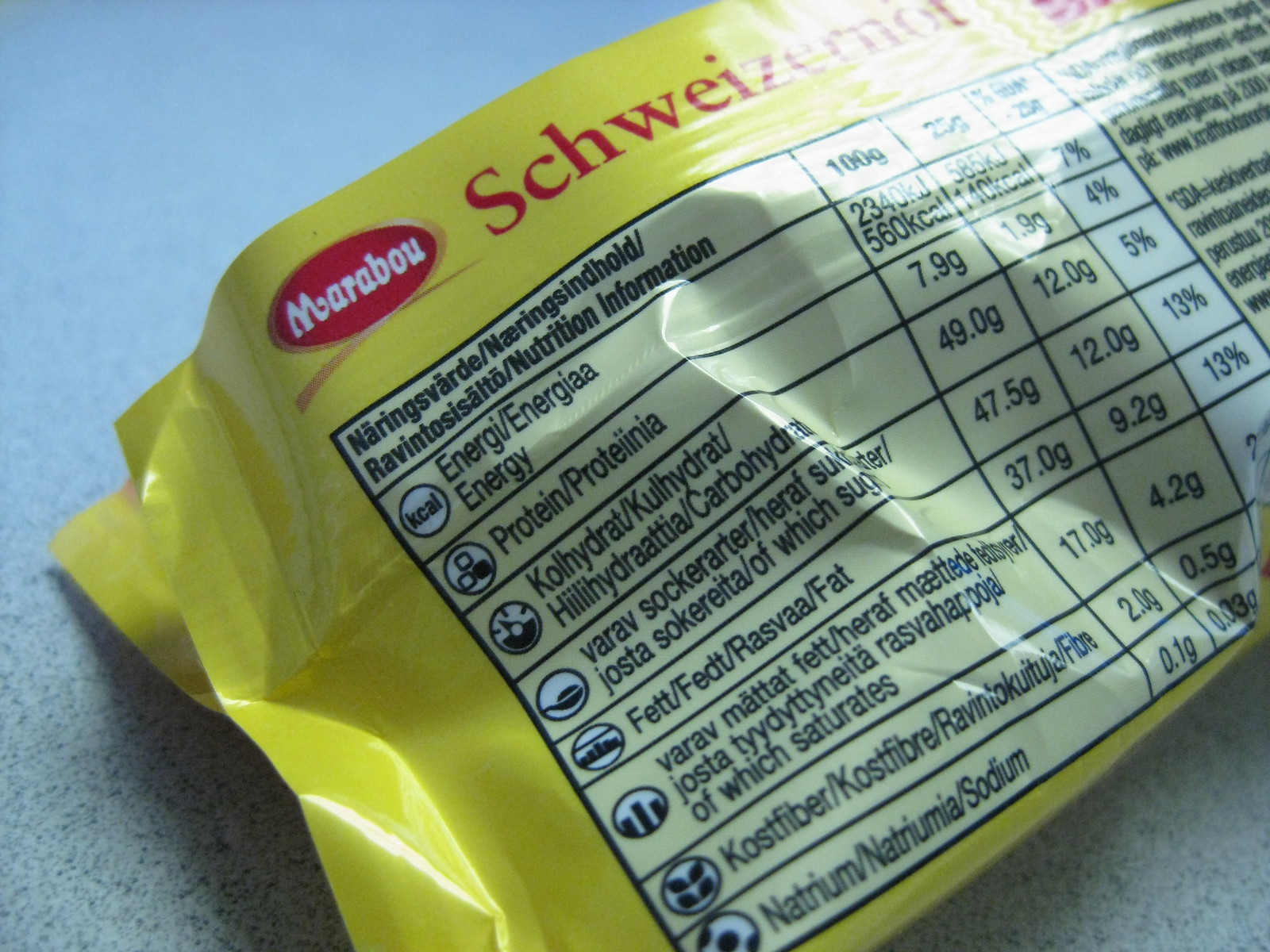The image showcases the back of a yellow food package labeled "Marabou Schweizernot," positioned on a speckled linoleum countertop with shades of gray and blue. The main visual feature is a red oval logo with white lettering that reads Marabou. Below the logo, there's a nutritional chart detailing information such as energy, protein, carbohydrates, sugars, fats, saturates, sodium, and fiber, with some parts in another language and some in English. The chart is organized within a white area bordered in black. The overall design consists of black text against a predominantly yellow background, with lighter yellow sections accentuating portions of the packaging.